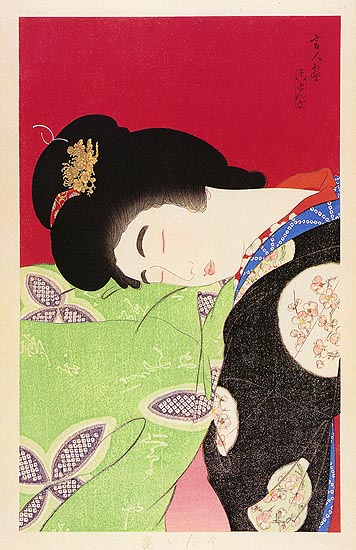This narrow vertical rectangular image depicts an Asian woman, potentially a geisha, lying her head down on her right side on what appears to be a table or surface with green fabric adorned with teardrop-shaped patterns and squiggly white lines. Her eyes are closed, and she exudes a serene, restful demeanor. The top of the image features a solid red background with vertical black symbols in a non-English language. The woman’s black hair is styled elegantly in an updo, decorated with a gold and red ornament. She wears a visually rich black kimono with intricate white floral patterns and large round symbols, a blue and red collar, and pink cuffs. The bottom portion of the image transitions to a light pale spring green background with purple leaf-like shapes. The overall piece is reminiscent of traditional Asian art prints, with a harmonious blend of colors and detailed adornments.